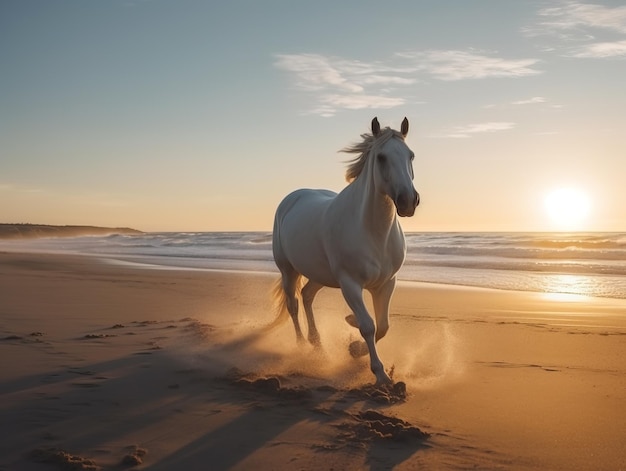In the foreground of this pristine beach photo, a majestic white horse with a shorter white mane and distinctive gray markings under its eyes and near its nostrils is running freely. The horse, captured from a front-right angle, kicks up a little dust from the smooth, tan-colored sand, leaving a trail of interrupted hoof prints that suggest a sudden direction change. The beach itself is serene with smooth, even sand except where the horse disturbs it. The shoreline blends seamlessly into the calm ocean, which features gentle waves with whitecaps rolling in towards the beach. The setting sun sits just above the horizon, casting a warm, golden light that mingles with soft pink and beige hues at the skyline. The sky is a clear, soft blue with scattered white clouds, and in the distance, the land curves and juts out slightly into the sea. This sunlit scene on a tranquil, clear day beautifully captures the spirit of nature and the unbridled grace of the horse.